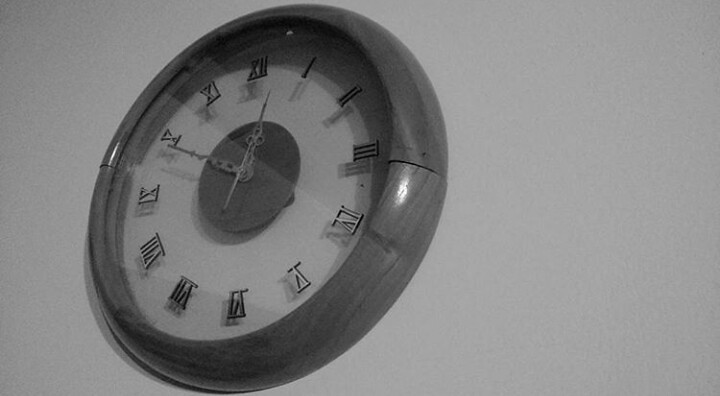This black-and-white photograph showcases a circular wall clock mounted on a pristine white wall. The clock features a wooden frame, with its natural wood grain texture subtly visible despite the monochromatic image. The timepiece is adorned with Roman numerals, providing a classic touch to its design. The clock's hands, thin and intricately crafted with delicate circular details, indicate the time is ten minutes to one. At the center of the clock, a large gray circle adds an elegant focal point to the overall composition.